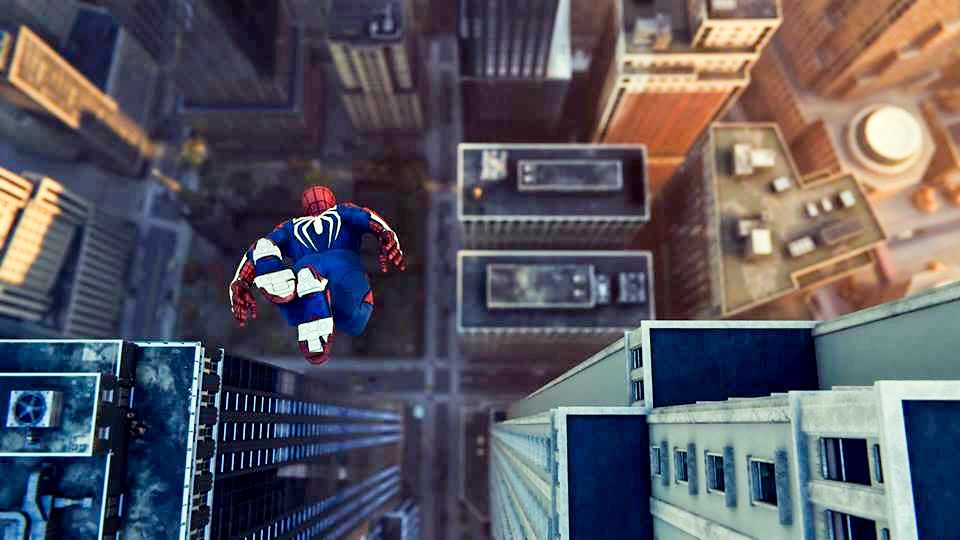The image appears to be a screenshot from a video game, depicting a dynamic aerial view of a cityscape from above. Central to the image is a figure diving towards the street level, clad in a predominantly blue one-piece suit. The suit features red and white gloves, along with a striking white spider emblem emblazoned on the back. The figure also wears a red helmet adorned with darker red stripes that coordinate with the gloves. The feet of the figure, although partially obscured, show four white blocks intersected by a blue stripe. The urban environment beneath is characterized by numerous flat-roofed buildings, adding to the metropolitan atmosphere of the scene.